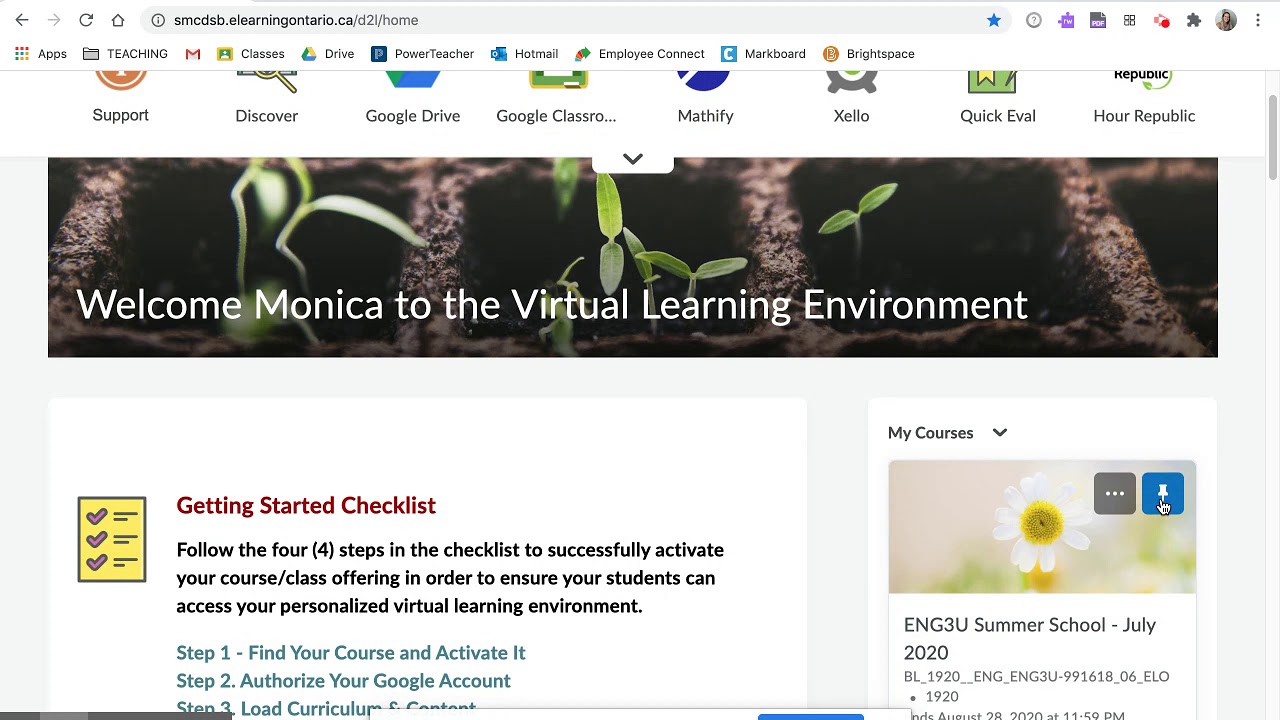The image showcases a well-structured webpage with a predominantly white background. At the topmost part of the page, there are navigation arrows—with the left arrow being active and the right one faded out, indicating it's unclickable. Following these is a series of iconic buttons: a refresh icon, a home button, a populated address bar, a blue star, a question mark within a circle, a purple puzzle piece resembling a disk, a user profile picture encased in a circle, and three vertical dots symbolizing a settings or options menu.

Moving downward, there is a menu listing various apps and tools, including Google Email, Classes, Drive, Power Teacher, Hotmail, Employee Connect, Mark Board, and Brightspace. Below this section, there is a partially covered banner with obscured icons.

Further down, the page features a footer with links labeled support, Discover, Google Drive, Google Classroom, Mathify, XELLO, Quick Eval, and "Our Republic" (phonetically spelled “H-O-U-R").

Additionally, there is a prominent close-up image of dirt featuring new seedlings or small sprouts—a visual metaphor for growth. Adjacent to this, the message "Welcome, Monica, to the virtual learning environment" is warmly displayed, accompanied by a "Getting Started Checklist." On the right side of the page, there is a dedicated section titled "My Courses," facilitating easy access to the user's enrolled classes.